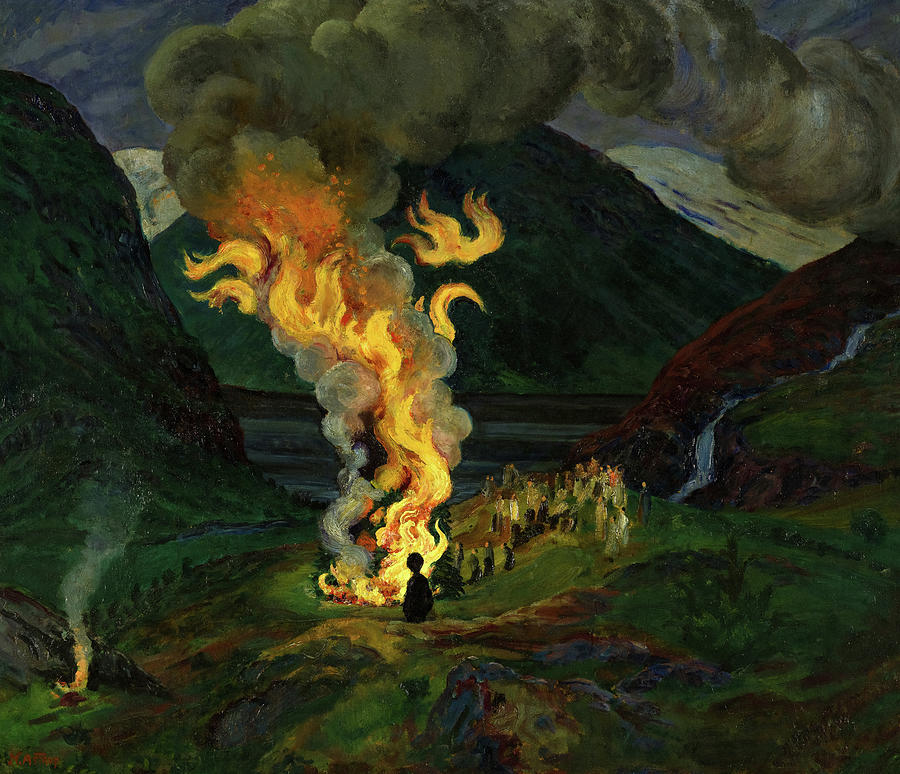The painting vividly depicts a dramatic scene set in the mountains under a dark blue sky. Dominating the center is a massive bonfire, its flames in striking hues of yellow, gold, and orange, reaching high into the sky—estimated to be around 25 to 50 feet. Dark, smoky tendrils waft from the top of the fire, drifting to the right. The surrounding environment includes a few green mountains and a bluish stream flowing downhill, adding a sense of life to the setting. Silhouetted against the blazing inferno, a group of people can be seen; one person sits while others stand, intently observing the towering flames. The entire scene is shrouded in thick, grayish smoke, creating a somber yet mesmerizing atmosphere around the gathering.